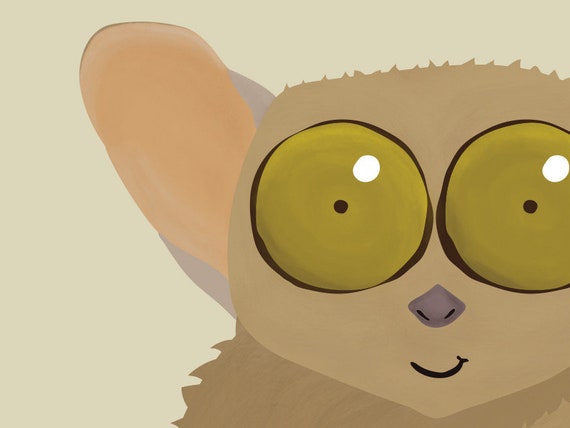This illustration depicts a cartoon character of a lemur-like animal, rendered in a digital watercolor style. The character's head dominates the image, set against a plain, matte green background. It has strikingly large, reddish-brown ears with peach insides, and enormous, vibrant green eyes complemented by tiny, dilated pupils. The creature's head features soft brown fur, which transitions to a darker brown on its neck. The animal has a small, gray nose and a delicate, black mouth drawn as a thin stroke to give the impression of a smile. The lemur appears slightly off-center, with only one of its large ears fully visible, contributing to the off-kilter but endearing charm of the illustration.